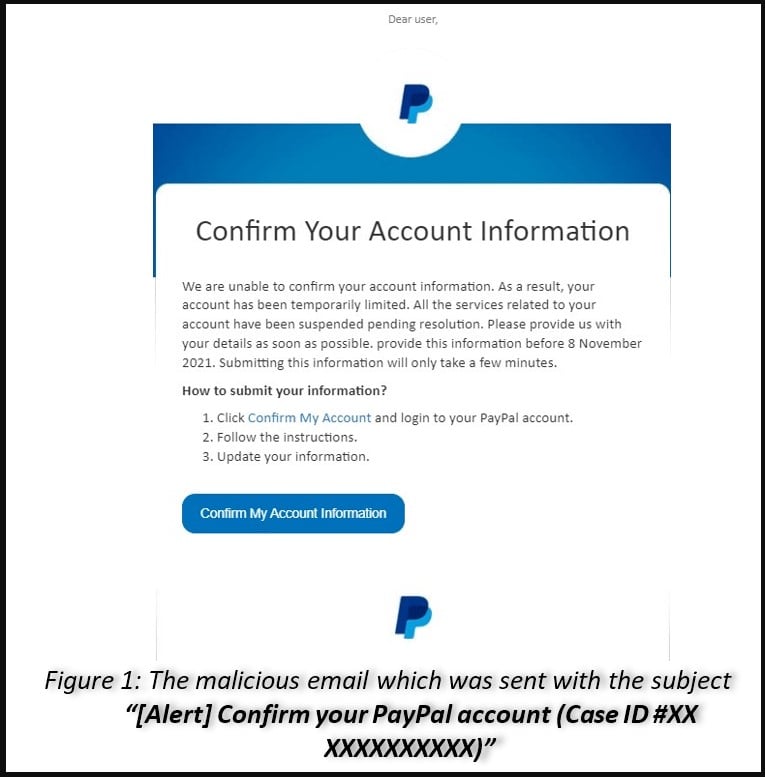The image is a vertically-oriented rectangle with a black border encasing it. It appears to be a phishing attempt mimicking a PayPal communication. At the top center, it begins with the salutation "Dear User," followed by the official PayPal logo featuring the two interlocking Ps. Below the logo is a blue banner that reads, "Confirm your account information."

In smaller text beneath the banner, the message states: "We are unable to confirm your account information. As a result, your account has been temporarily limited. All services related to your account have been suspended pending resolution. Please provide us with your details as soon as possible. Provide this information before 8th of November 2021. Submitting this information will only take a few minutes."

The instructions section is next, explaining how to resolve the issue:
1. Click "Confirm my account" (this text is blue and clickable) and log in to your PayPal account.
2. Follow the on-screen instructions.
3. Update your information.

A blue, oblong button underneath reads, "Confirm my account information" in white text.

Towards the bottom of the image, the PayPal logo appears again, accompanied by the larger text: "Figure 1: The malicious email which was sent with the subject 'Alert: Confirm your PayPal account.'"